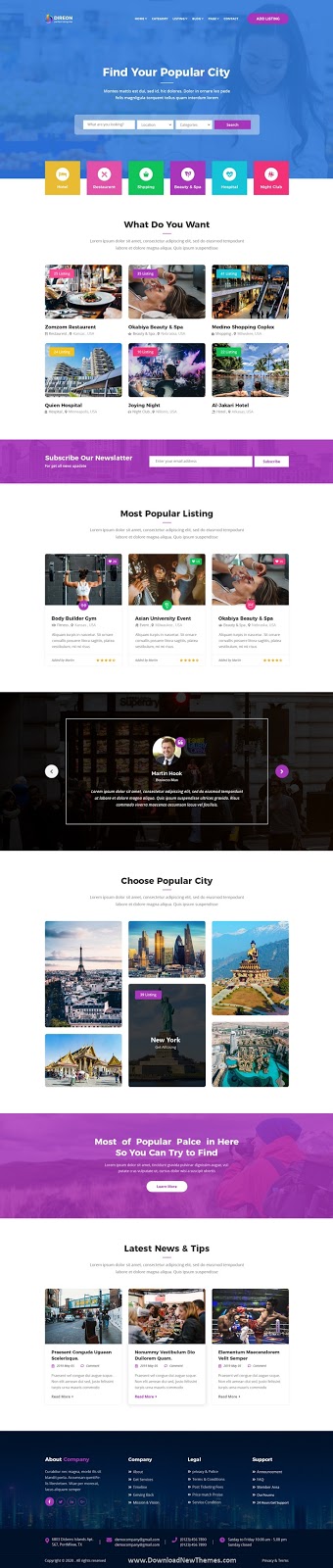This image depicts a webpage with a notably low-quality resolution, making it quite blurry and difficult to read due to the small size of the text. At the top center of the page, the phrase "Find Your Popular City" is visible. Directly beneath this header, there are three search bars aligned horizontally. Further down, the text "What do you want" is prominently displayed in black. Below this text, the layout contains six different images arranged in two rows: two images on the left, two in the middle, and two on the right. 

The top-left image showcases a dish of food on a plate, while the adjacent top-right image features a woman lying down. Continuing downward, the section labeled "Most Popular Listings" is evident, followed by three distinct sections. The leftmost section contains the image of a person.